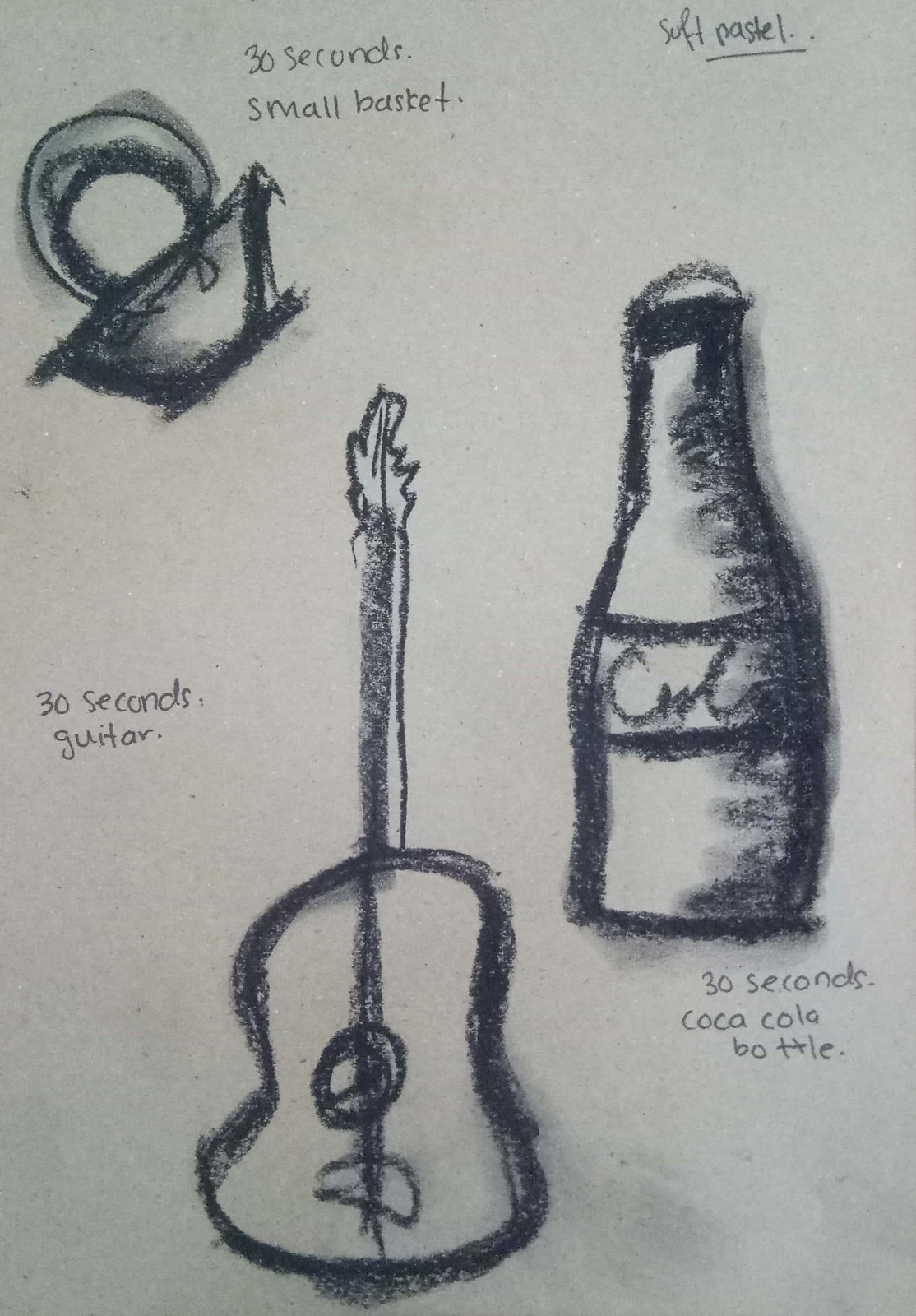The image features three intricate charcoal drawings on a piece of white paper, focusing on the themes of quick-rendered sketches seemingly for an art project. The primary label "30 seconds" is prominently reiterated throughout, implying these are rapid sketches. On the upper left, there is a black and white drawing labeled "30 seconds small basket," which resembles more of an abstract or stylized basket, almost looking like a cereal bowl with a plate partially inserted into it. In the middle left of the page, another label reads "30 seconds guitar." This drawing depicts a guitar with an acoustic body and an electric guitar head, rendered in thick, smudgy black charcoal lines. Finally, on the lower right portion of the paper, the label "30 seconds Coca-Cola bottle" accompanies a charcoal sketch of a classic Coca-Cola glass bottle, detailed with horizontal stripes and the word "Cola" between them. The top right corner of the drawing has the underlined text "soft pastel," marking it clearly as part of an art exercise. Overall, the artwork combines a blend of stylization and raw, rapid sketch techniques, portraying everyday objects with a unique, hurried touch.